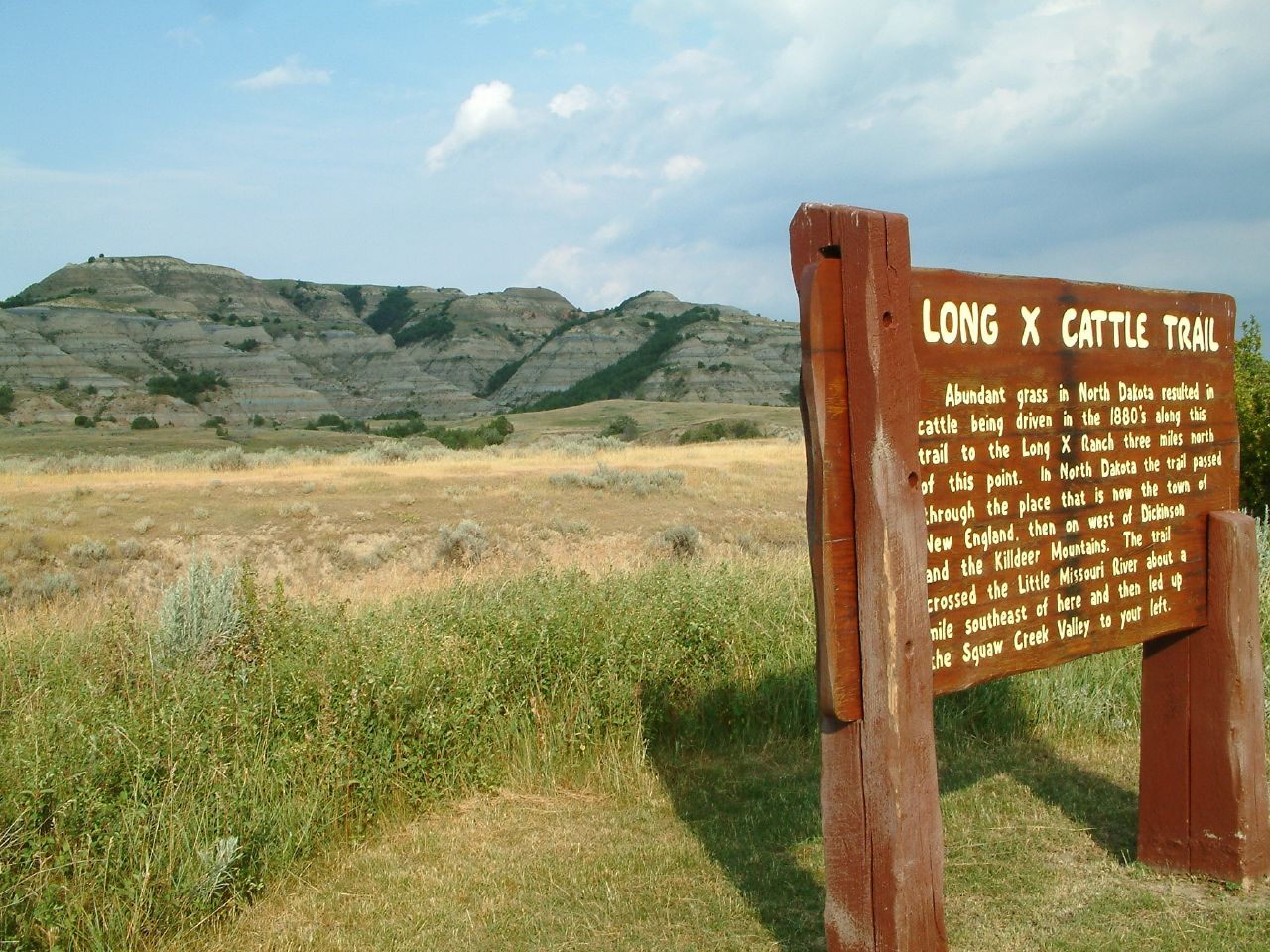This image captures a historical wooden sign for the Long X Cattle Trail situated in the midst of breathtaking natural scenery on a bright, sunny day with a few fluffy clouds in the background. The foreground features a wooden sign, brown in color with white lettering, detailing the trail's historical significance: "Abundant grass in North Dakota resulted in cattle being driven in the 1880s along this trail to the Long X Ranch, three miles north of this point." The sign narrates how the trail passed through what is now the town of New England, then west of Dickinson and the Kildare Mountains, crossed the Little Missouri River about a mile southeast of there, and led up the Squaw Creek Valley to the left. Surrounding the sign are flat fields with patches of brush, bushes, green grass, sand, and tumbleweeds, under a clear blue sky adorned by both bright sunlight and a few clouds. Towering mountains, which could be part of the rocky Badlands, dominate the majestic background. The image is devoid of people, creating an untouched and historically immersive scene highlighted by the vivid colors of the landscape: blue, gray, green, brown, and tan.